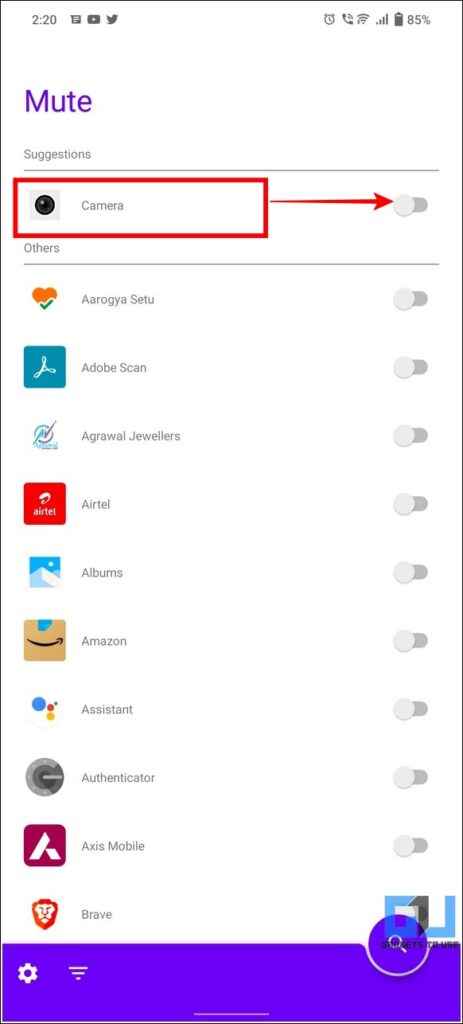The image displays a vertical format resembling a smartphone interface featuring multiple app icons. At the top left, the time is displayed as 2:20, accompanied by a YouTube icon, Twitter icon, and message icon. The top right corner includes various status indicators: a clock, an 85% charged battery with its symbol, a Wi-Fi symbol, and a phone icon. Additionally, "mute" is displayed in purple text at the top left, followed by the word "Suggestions" underneath a gray line.

Below, the word "Camera" appears beside a camera icon, both highlighted by a red box outline with an arrow pointing towards a gray button. Proceeding down, there is a section titled "Others," with a list of various apps: "Arogya Setu" accompanied by a heart icon, "Adobe Scan" with a blue square icon, "Agrawal Jewelers" with an unidentified icon, "Airtel" represented by a red square, "Albums" featuring a mountain icon, "Amazon," "Assistant," "Authenticator," "Access Mobile," and "Brave," identified by a lion's face on a shield. Each app name is associated with unchecked buttons. 

At the bottom of the screen, a purplish area features a prominent circular icon with a white magnifying glass inside, indicating a search function.